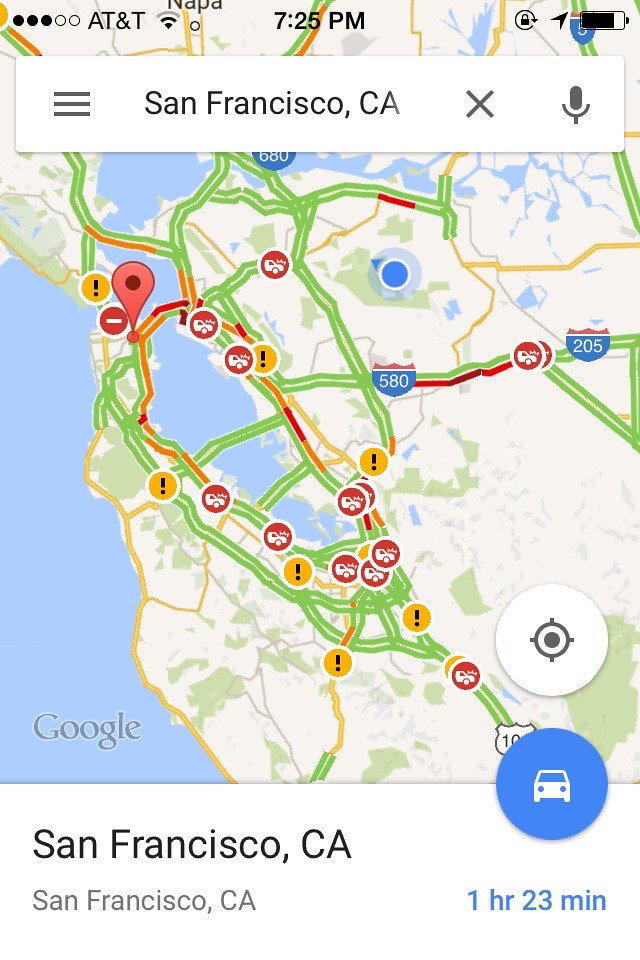This image is a screenshot of Google Maps taken from a mobile device. The top section of the image includes various mobile icons: on the left, it shows the AT&T carrier name, a Wi-Fi symbol, and the time displayed as 7:25 PM. On the right, there's a battery icon indicating around 25% charge. Below this, a white bar states "San Francisco, California" with an 'X' to close the search and a microphone symbol for voice commands.

The map itself focuses on San Francisco, California, highlighting various road conditions with green, yellow, and red lines, indicative of traffic flow. There are numerous icons, including red pins, yellow circles with black exclamation points indicating warnings or traffic issues, and symbols representing cars and potential car accidents. The user's current location appears to be quite far from the destination pin, visible on the right side of the map. The bottom left corner displays the Google logo, while in the bottom right, it indicates a travel time of one hour and 23 minutes to the pinned location, signified by a blue circle with a white car icon inside it. The map background features blue water contrasting the white land area, enhancing the geographical details of the city.